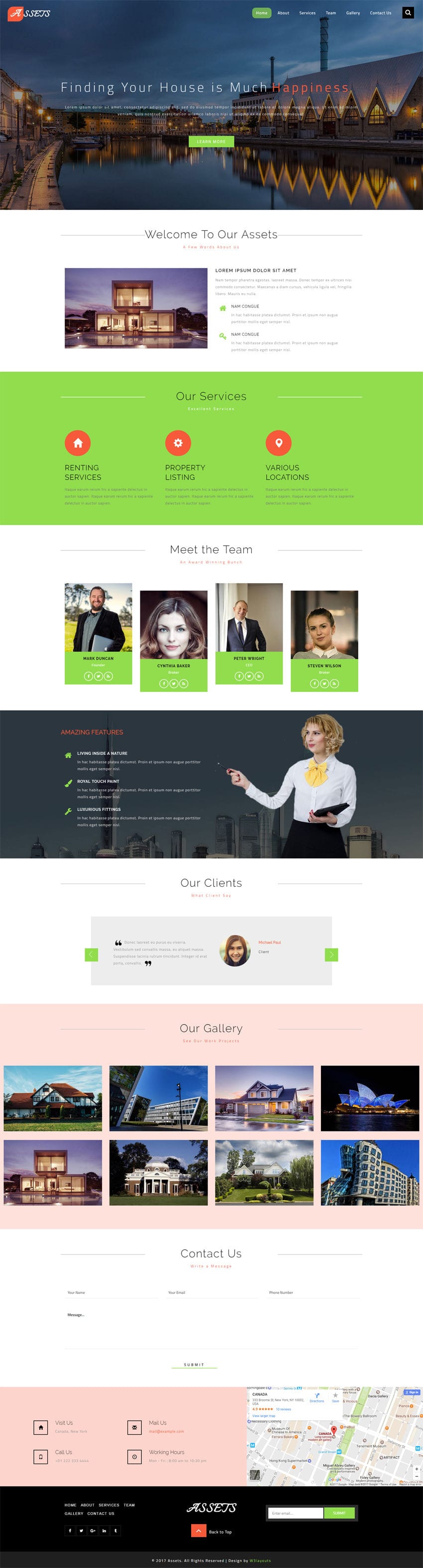The image features a picturesque scene at the top, showcasing a river or lake surrounded by buildings. The sky and water are predominantly blue, creating a tranquil atmosphere, while the buildings exhibit a range of brown hues. Above the main scene, there is a red rectangle containing some text, accompanied by additional white text adjacent to it.

Below this, a green rectangle stretches to the right with accompanying white text. Further down, a black rectangle appears, though its contents are indistinguishable. Centered on the image are a series of words, predominantly in white, with the final word in red; some text is too small to be legible.

Continuing downward, there is another green rectangle underlined with a line, followed by more text and another underline. Accompanying these elements is an image resembling a house with text to its right. Another green rectangle below this features a red oval with illegible content; in total, there are three red ovals with different symbols and text both above and below them.

Subsequently, there are four individual pictures of people, each with a green rectangle beneath them containing text. Below these lies a large, blackish-gray rectangle marked by red text, green symbols, and white text. To the right of this rectangle is the image of a woman, bordered by faint gray lines with accompanying text.

Further along, a gray rectangle is flanked by green squares, each containing writing. A circular emblem with a face and adjacent text follows, succeeded by a pink rectangle with some text at the top. This section includes eight images depicting various landscapes, houses, or apartment buildings, surrounded by faint gray lines with additional accompanying text.

Beneath this portion is more text, followed by another pink rectangle containing four squares with indiscernible symbols and adjacent text. On the right side, a map is included, and below it, a black rectangle features white text, alongside inner red and green rectangles.